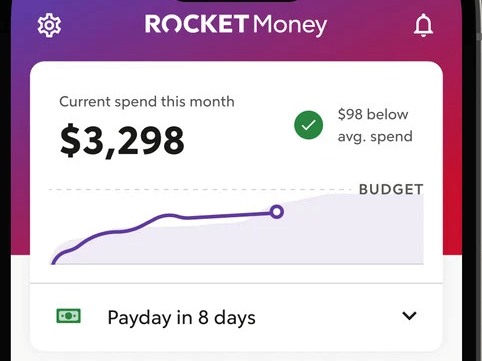In this image capturing the screen of someone's phone, the user is viewing the Rocket Money app. At the top of the screen, "ROCKET" is prominently displayed in all capital white letters, except for the 'O,' which has a distinctive chunk missing from its bottom. Adjacent to this, "Money" is written with a capital 'M,' followed by lowercase letters. The left side features a white gear icon, while the right sports a white bell icon. 

The background transitions from a purplish hue at the center to pink and then red towards the right. Below this, a rectangular box displays "Current Spend This Month" in black bold text. Below this, in larger bold text, it shows "$3,298," accompanied by a white check mark inside a green circle, and the text "$98 below average spend" displayed underneath.

Further down the interface, the user's budget information is illustrated with a purple line tracking along a lighter purple zone. Accompanying this visual is the word "budget” along with an alert indicating "payday in 8 days."